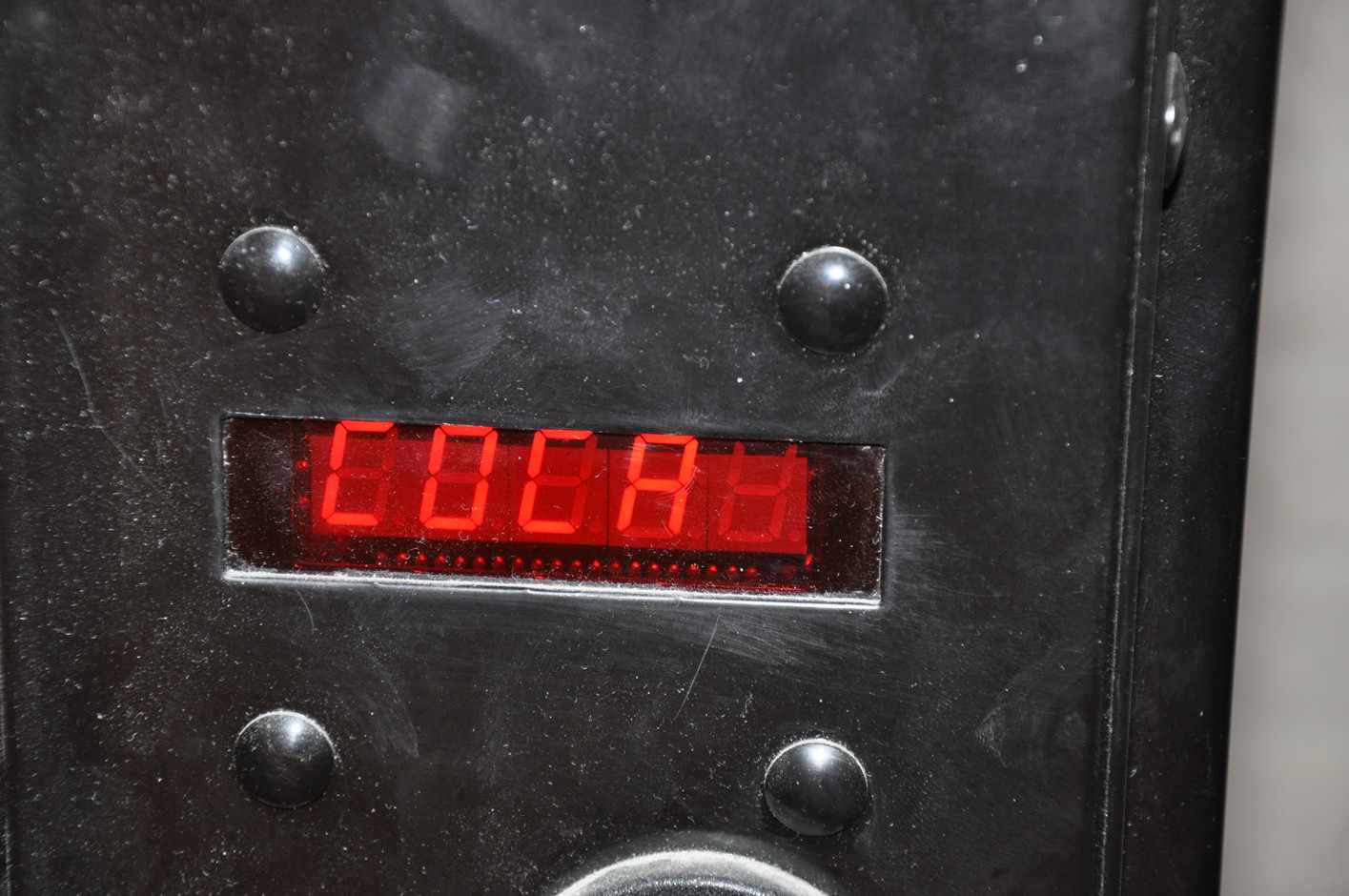The image features a vertically-oriented, black metal machine with a glossy enamel finish, though it appears dusty and well-used. Prominently, there is a bright red digital display in the center of the machine, covered by a red glass screen. The display shows five digits, which are currently all lit up as eights, though the exact numbers are difficult to discern due to the lighting. Surrounding the digital display are four smooth bolts, with two positioned on each side, securing the red screen to the machine.